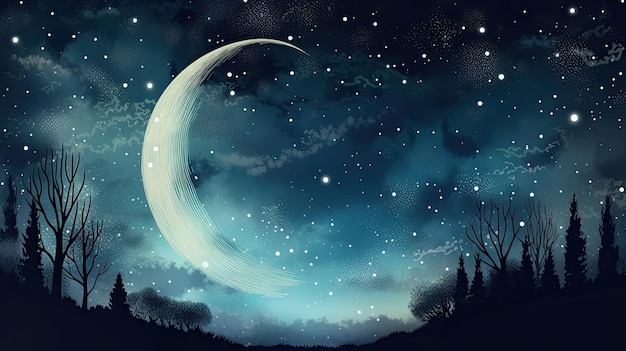This illustration portrays a melancholic night sky dominated by a large crescent moon that almost looks like a cream-colored paint stroke. The sky exhibits a gradient ranging from a nearly black hue at the top to dark blue and lighter blue shades, interspersed with cloudiness. Numerous white circles, representing stars, are scattered across the sky, with some seemingly positioned in front of the moon. Adding to the eerie atmosphere, the clouds on the right form an ominous face. Silhouetted along the bottom left and bottom right edges, a variety of trees, including triangular evergreen pines and bare, leafless branches, emerge from a slightly hilly terrain. These trees are portrayed in black, emphasizing the darkness of the scene, while grayish clouds linger at the very bottom, enhancing the overall mysterious and haunting ambiance.